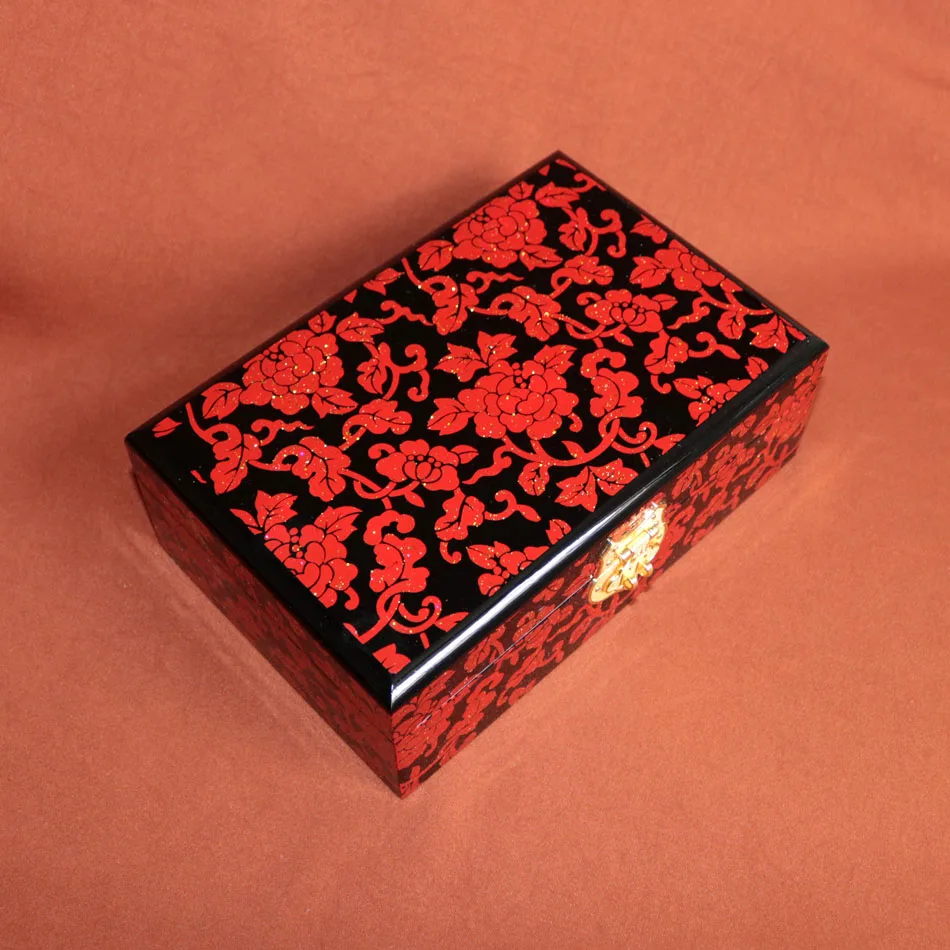The photograph features a rectangular lacquered jewelry box, captured from an aerial view on a salmon-pink or rust-colored background that appears to be either cloth or paper. The box is primarily black, adorned with an intricate pattern of red flowers, looping vines, and leaves. These embellishments, including red petals and possibly bunches of grapes, are highlighted with subtle gold flecks. A prominent gold clasp is situated at the front, connecting the top and bottom sections. The lacquer's sheen creates a harsh highlight on one edge of the box and the clasp, slightly obscuring the clasp’s details.